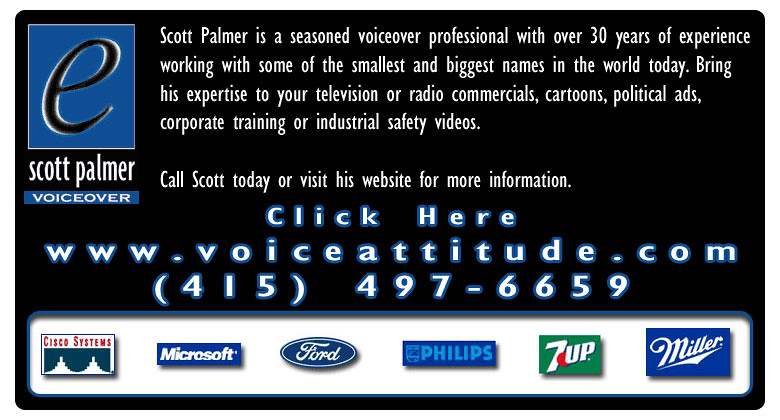The advertisement for Scott Palmer's voiceover services is set against a black background in a horizontal rectangle. In the top left corner, there is a logo of a black letter "E" within a blue square. Beneath this, it says "Scott Palmer" in white letters, followed by "Voiceover." To the right of the logo, in large white text, it reads: "Scott Palmer is a seasoned voiceover professional with over 30 years of experience. He has worked with some of the smallest and biggest names in the world today. Bring his expertise to your television or radio commercials, cartoons, political ads, corporate training, or industrial safety videos." 

Underneath this text, there is a call to action in the same white font: "Call Scott today or visit his website for more information." Following this, in white print outlined in blue, it says "click here" in large letters. Below this directive, the advertisement lists a web address and a phone number, both in large white letters outlined in blue.

At the bottom of the rectangle, there is a white box featuring the logos of companies Scott Palmer has worked with, including Cisco Systems, Microsoft, Ford, Philips, 7-Up, and Miller.